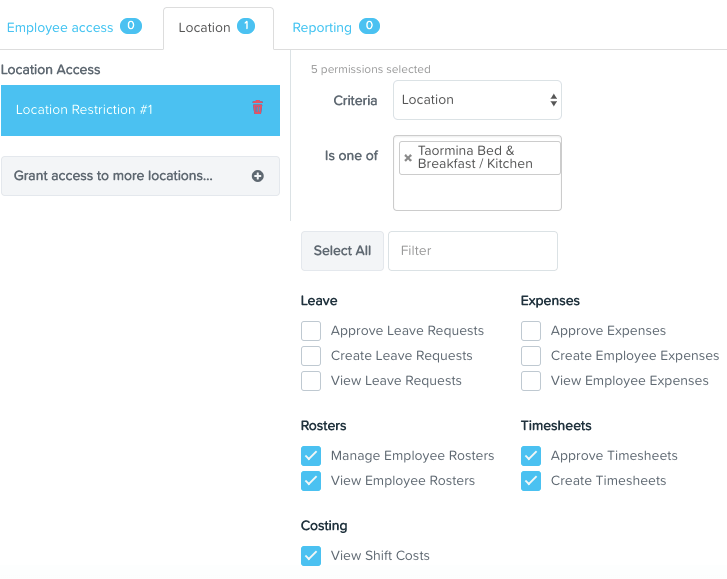**Detailed Caption:**

The image is a screenshot of an HR application interface, showcasing various tabs and sections related to employee and location access management. At the top of the interface, there are three tabs:

1. **Employee Access:** This tab is labeled in blue on the left and contains a blue oval with the number “0” in white.
   
2. **Location:** The currently selected tab, displayed in white text on a black background, also has a blue oval with the number “1” in white.

3. **Reporting:** An unselected tab in blue text, which also contains a blue oval with the number “0” in white.

On the left side of the screen is a section titled "Location Access" in black. Below this is a blue horizontal rectangular button with white lettering that reads "Location Restriction 1". Adjacent to this button on the right is a red trash can icon. Below this button, there is a gray bar that reads "Grant access to more locations" in black text, with a gray circle containing a white plus sign on the right side.

On the right-hand side of the interface, in a white section, it is noted that "5 Permissions Selected." Directly to the left of a dropdown selection box, there is the label "Criteria" with the selected entry being "Location." The subsequent line reads "is one of," followed by search filters comprising "Taormina Bed and Breakfast / Kitchen". Below this line, a white button with black lettering indicates "Select All," accompanied by a section labeled "Filter" on the right.

The interface then displays various permissions organized into categories:

- **Leave:** Featuring three unchecked checkboxes labeled "Approve leave request," "Create leave request," and "View leave request."

- **Expenses:** Includes three unchecked white checkboxes labeled "Approve expenses," "Create employee expenses," and "View employee expenses."

- **Rosters:** Displays two blue checkboxes with white checkmarks, labeled "Manage employee rosters" and "View employee rosters."

- **Timesheets:** Contains two blue checkboxes with white checkmarks, labeled "Approve timesheets" and "Create timesheets."

- **Costing:** The final section is titled "Costing" in bold black text and includes a blue checkbox with a white checkmark labeled "View shift costs."